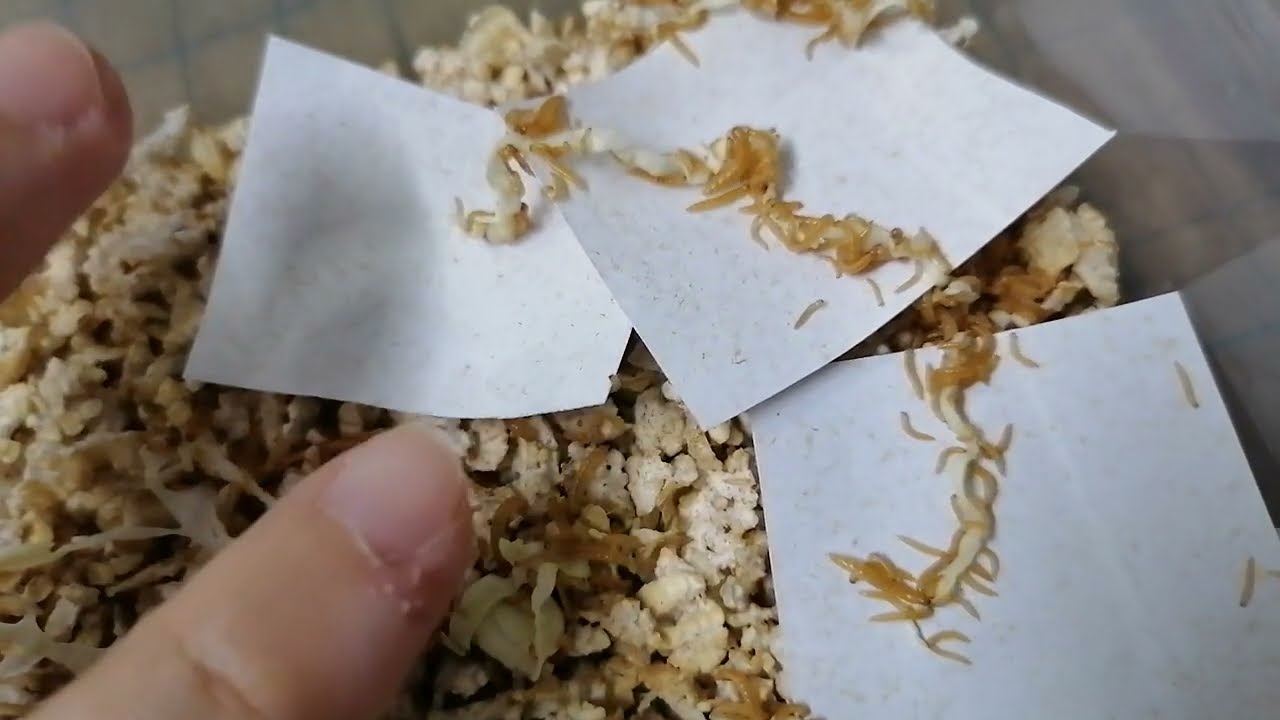The image is a close-up photograph featuring a hand holding three small squares of white paper, each scattered with an orange-brown organic material that resembles crushed herbs or potpourri. The papers rest atop a bed of similar organic material, which might be a rice cake, crushed herbs, or possibly dirt. The hand, which extends from the left side of the image, is notable for its chipped and possibly bruised fingernails, with one finger showing signs of a bloody scrape. The background is white, and the lighting casts some shadows, emphasizing the texture and color variations of the organic material.